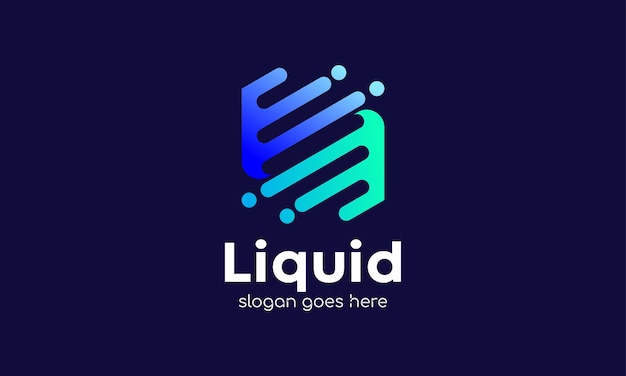This image features a logo template on a dark brown rectangular background, designed for a company named "Liquid." The logo's main design element consists of interconnected lines and dots that evoke the appearance of water. It employs a gradient color scheme that transitions from teal to blue, providing an aqua-like effect. Above the gradient lines, there are two distinct sets of three lines each—one set is blue, and the other is aquamarine—interspersed with four dots at their ends. The lines run in opposite directions and are connected, creating a visually appealing, abstract water motif. Below the logo design, the word "Liquid" is displayed in white sans-serif font, with an uppercase "L" followed by lowercase letters. Directly beneath this, in smaller white text, the placeholder slogan "slogan goes here" is written, also in a sans-serif font. This template appears to be intended for potential sale or as part of a portfolio, where buyers can customize the name and slogan to fit their needs.